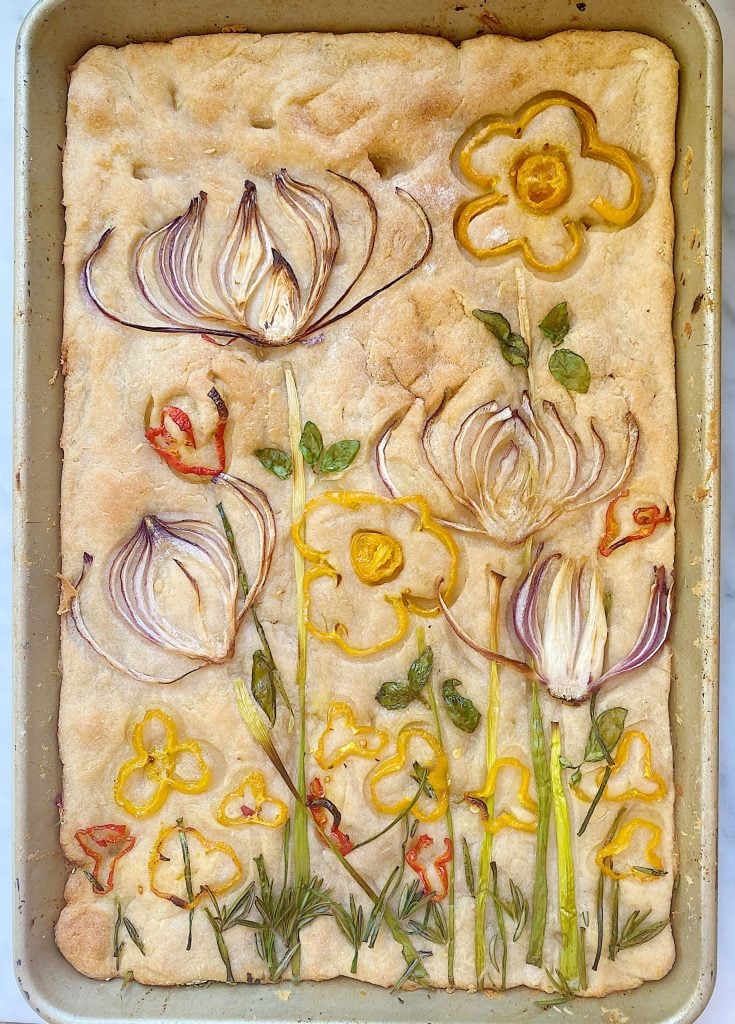This image showcases a top-down view of a beautifully decorated rectangular cake or pastry in a metal baking pan. Vertically aligned, the pan displays an intricately designed masterpiece that resembles a delicate painting. The baked good, lying golden brown around the edges and beige in the center, serves as the canvas for this edible artwork. 

Finely piped flowers in shades of purple, white, yellow, and delicately portraying stems and leaves fill the entire surface, creating a captivating floral arrangement. Among the flowers, meticulously created to resemble daisies and orchid-like blossoms, are smaller yellow daisies beneath and various green elements such as chives mimicking stems, and herbs like mint leaves, thyme, and rosemary that add to the leafy appearance. Sliced onions artfully crafted to resemble flowers, along with thinly cut red and yellow bell peppers, further enhance the texture and realism of this decorative display. This creation, reminiscent of a museum-quality piece, exemplifies a light touch and detailed craftsmanship, transforming an ordinary baked good into a stunning, edible work of art.